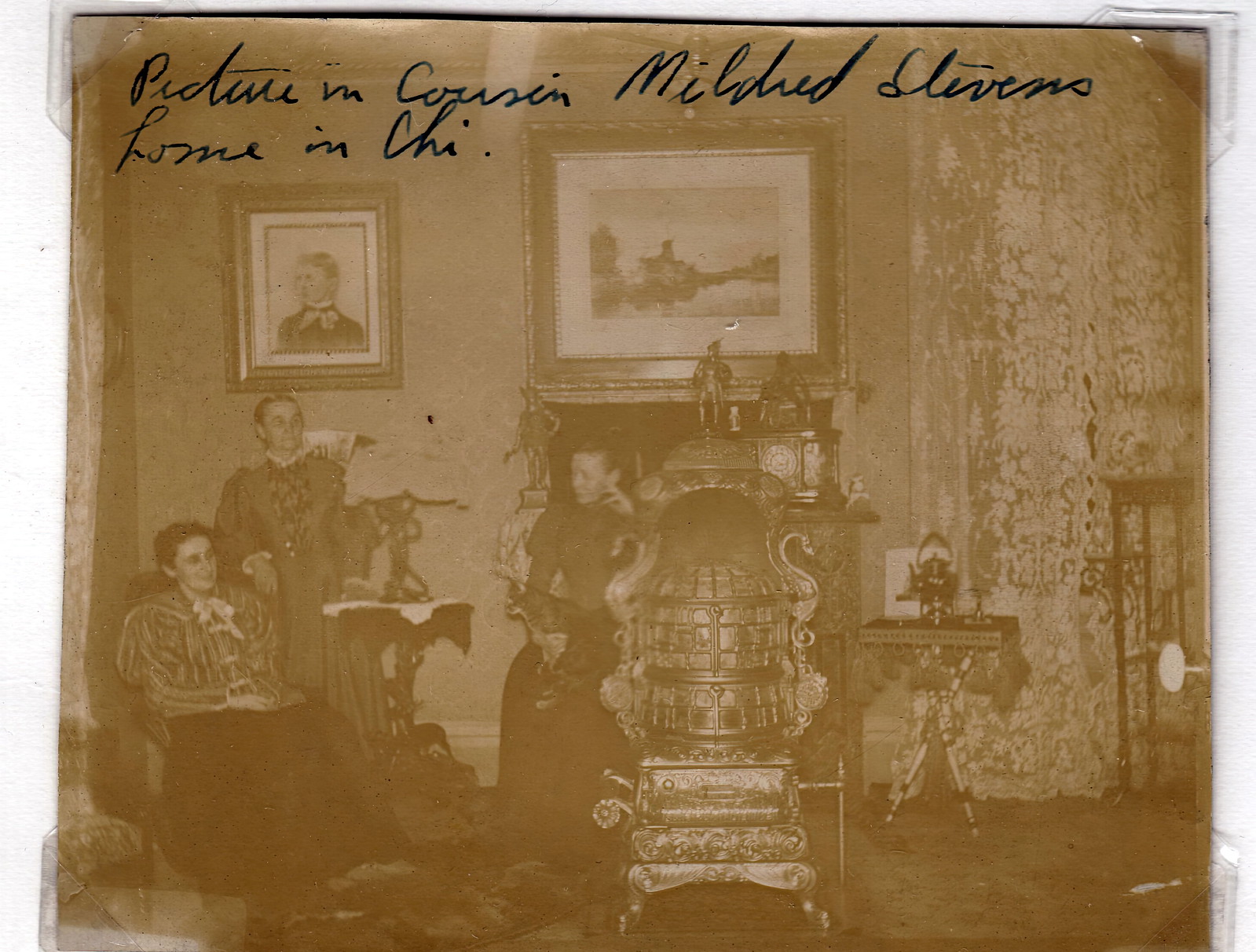This photograph is an old, faded image that appears to have transitioned from black and white to sepia tones over time. The right side of the photo shows signs of possible water damage. The image is set within a photo album, indicated by clear plastic corner holders. Handwritten in messy black cursive at the top of the photograph, it reads "Picture in Cousin Mildred Stevens' Home in CHI," likely referring to Chicago.

The setting is a dilapidated living room with white lace curtains that add a touch of faded elegance. The wall in the background shows signs of deterioration. Central to the image, there is a stove or furnace. Three Caucasian women dressed in old-style Victorian gowns are seen in the room; one woman stands while the other two are seated. Above them, two framed photos adorn the wall—a portrait of a man on the left and a landscape or river scene in the center. To the right side of the room, a table is also visible.